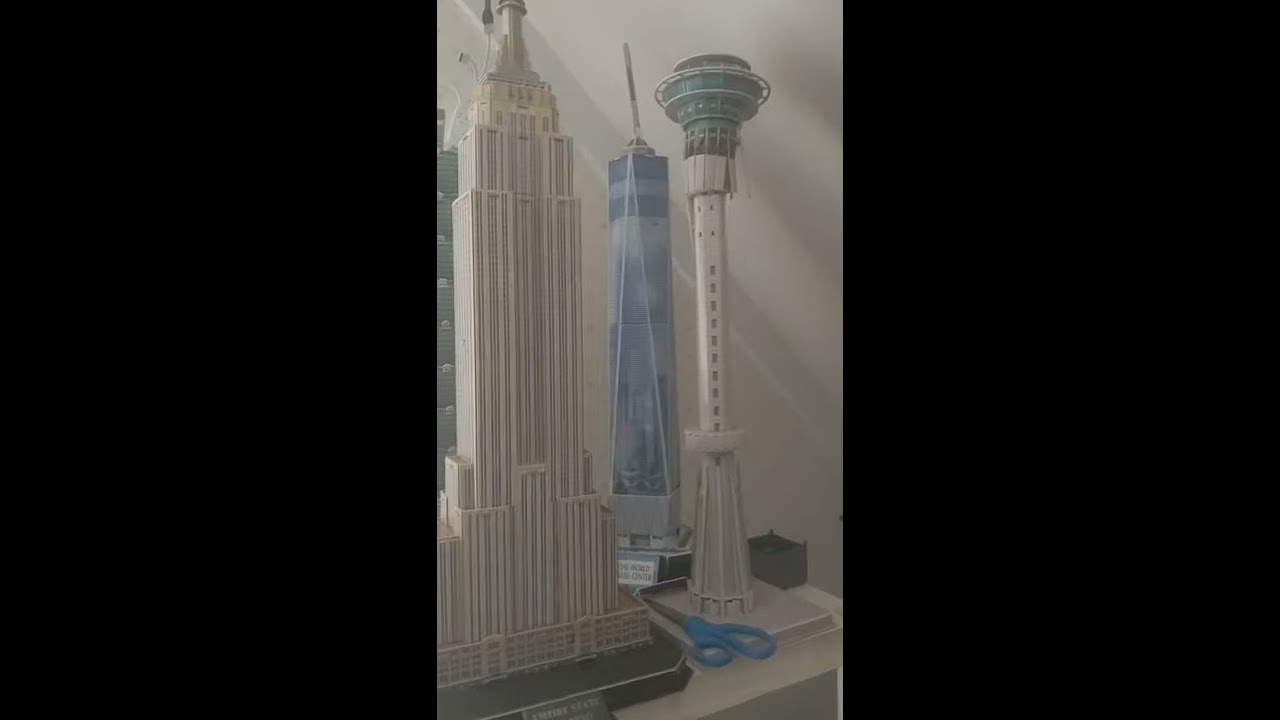The image depicts an artistic drawing rendered digitally, portraying three prominent architectural models situated on a table. The left-most building resembles the Empire State Building, characterized by its light tan color and iconic spire. The central structure appears to represent One World Trade Center, distinguished by its light blue and grayish-blue tones. To the right, a slender tower evokes the Space Needle or a similar revolving tower, marked by its white hue and grayish-blue support. A pair of blue-handled scissors rests between the Empire State Building and the right-most structure. The composition occupies the central third of the frame, flanked by black margins on both sides. The background features a monochromatic wall with varying shades of gray, devoid of any additional elements. The scene resembles a diorama or a creative rendering within an art studio, emphasizing the intricate details and colors of the buildings against a stark, minimalist background.